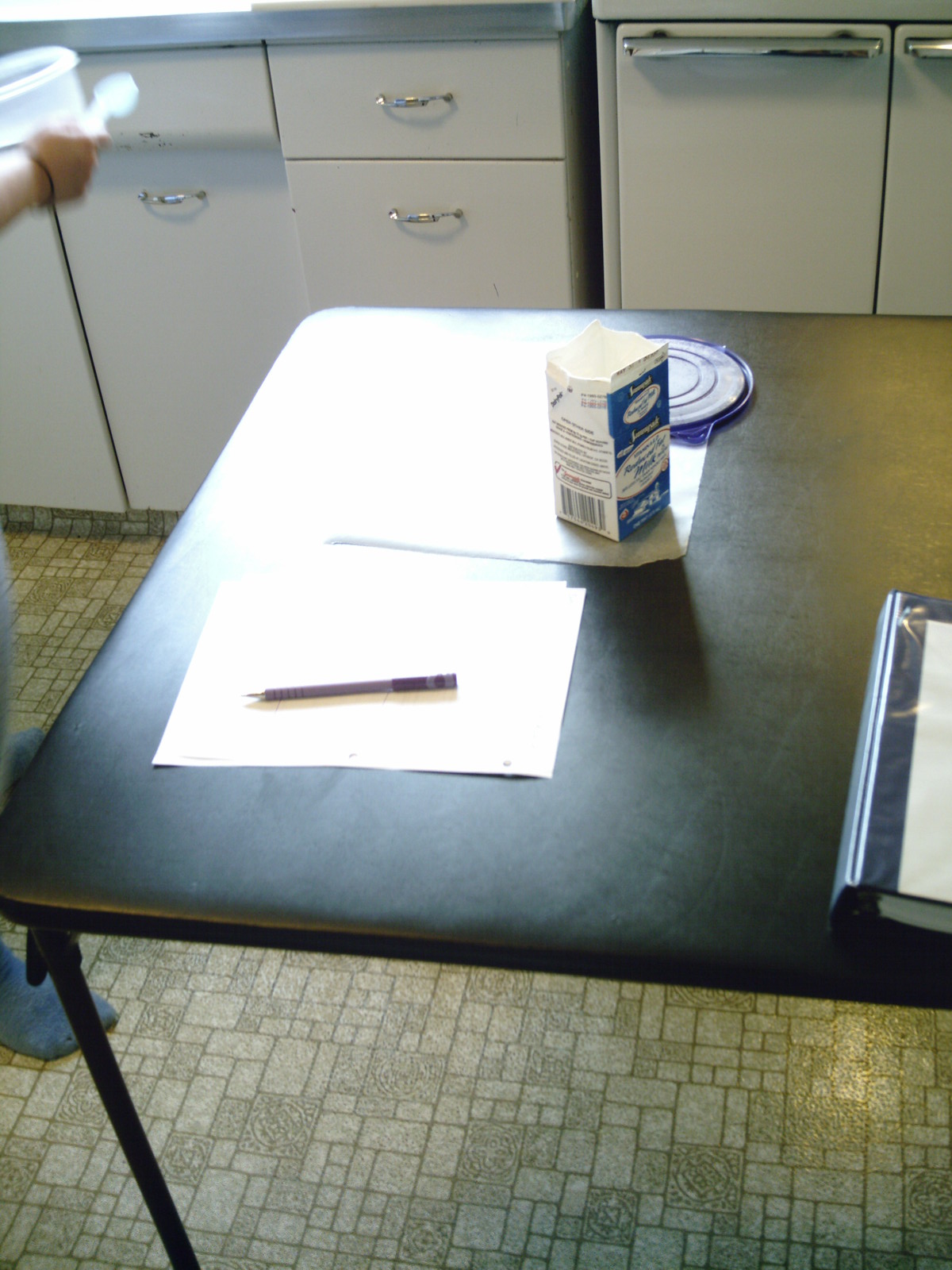In this photo, a bustling kitchen scene unfolds. The room features brownish gold tile flooring and stark white cabinets in the background, indicative of a typical home kitchen setup. Dominating the center of the image is a black card gaming table, cluttered with various pieces of paper illuminated by sunlight streaming in from an unseen window. The bright light obscures any text that might be on the papers. A school-style milk carton, torn open at the side, sits prominently on the table. Behind it, a lid belonging to a container held by someone can be seen. In the far left corner, the feet of an individual standing on the tile floor are partially visible. Another person is captured in blurred motion, holding a spoon and walking towards the sink; they are likely the owner of the container lid on the table. To the far right, a binder filled with papers lies closed, with its contents remaining a mystery.